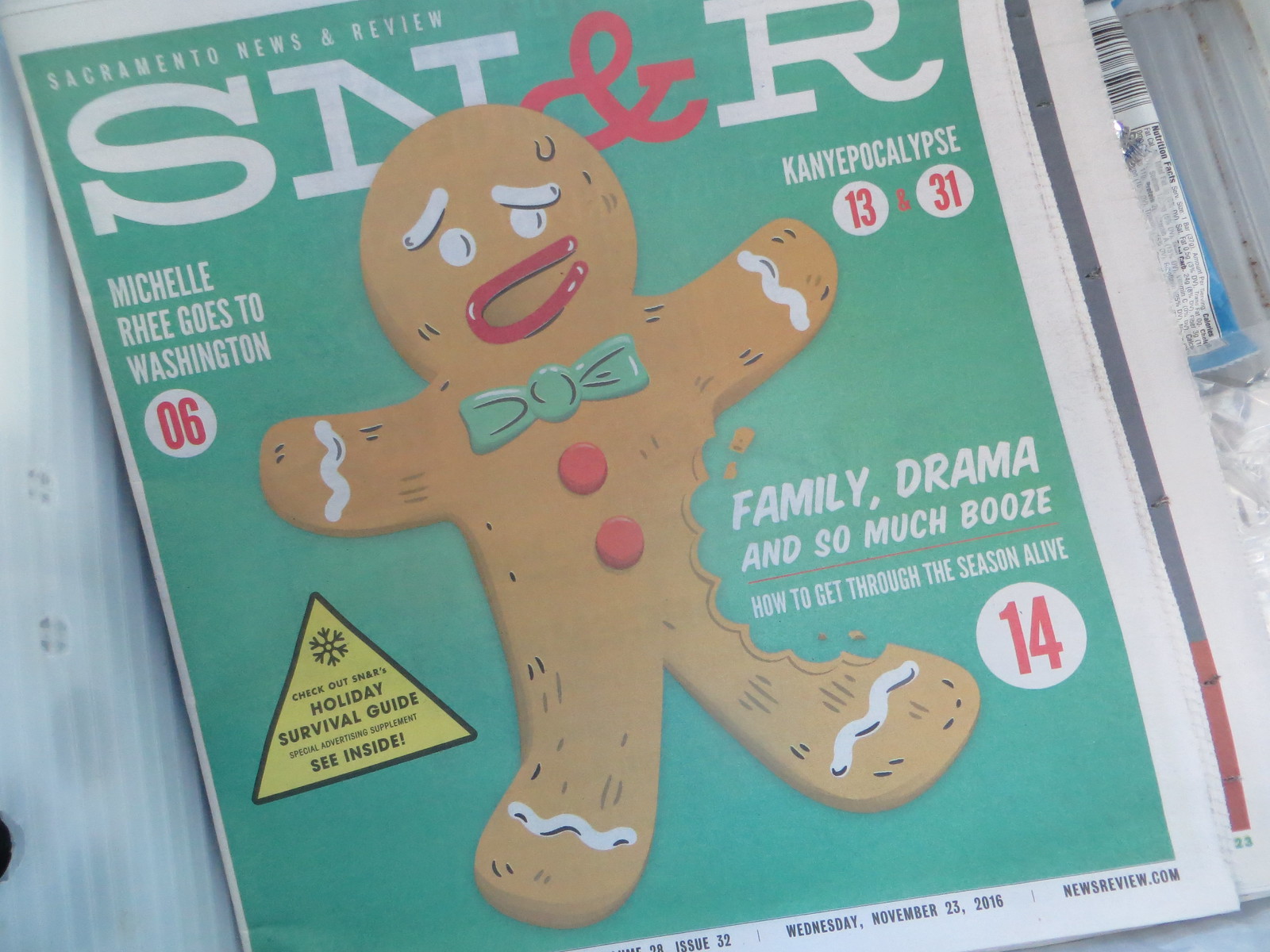This is a cover of the Sacramento News & Review from November 23, 2016, featuring a holiday-themed design. At the center of the cover is a brown gingerbread cookie with a bite taken out of its left side, adorned with a light green bow tie, red lips and buttons, white eyes, eyebrows, socks, and details on its arms. Surrounding the gingerbread cookie are various article titles in white text. At the top, "SNNR" is prominently displayed in large white letters with a red "N" symbol. The left side of the cover features the headline, "Michelle Rhee Goes to Washington." Below this, and beneath the gingerbread's left arm, is a triangle label with the text "Holiday Survival Guide: See Inside," alongside another headline, "Family Drama and So Much Booze: How to Get Through the Season Alive." To the right of the gingerbread, under the letter "R" from the title, the text "Kanye-pocalypse" stands out. The cover also mentions that the issue includes a special advertising supplement and directs readers to newsreview.com. The background color of the cover is light green, enhancing the festive atmosphere of the design.